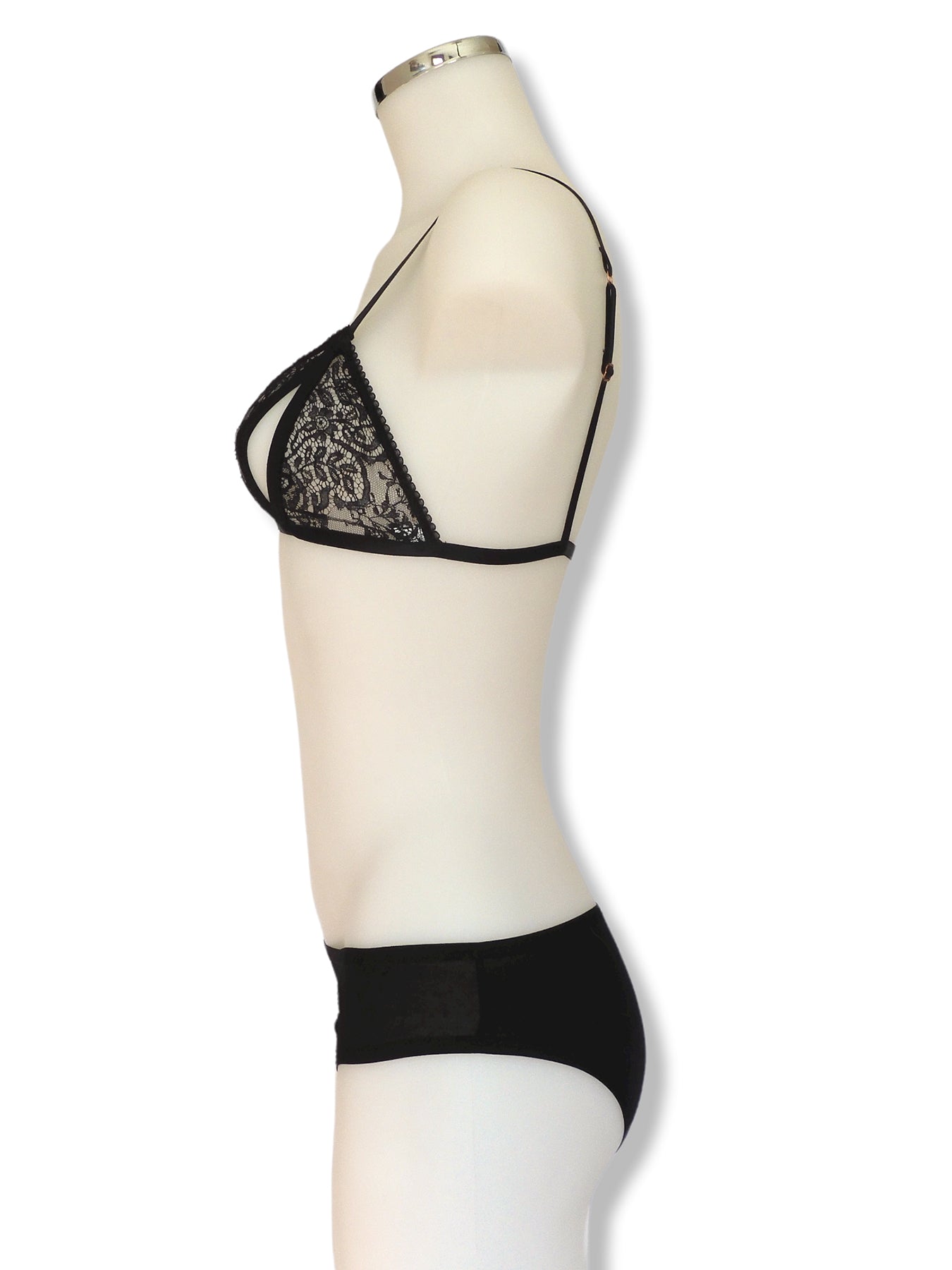This detailed image captures the side profile of a smooth, white plastic mannequin set against a stark white background. The mannequin, which is devoid of a head and arms, features a silver cap where the head would typically be. It is turned to the left, showcasing its elegant form. The mannequin is adorned in a black lacy bra with thin straps and a floral pattern, accentuating its delicate design. The lace bra is notably see-through, with a thin band wrapping around to hook at the back. Complementing the bra, the mannequin also wears black bikini-style panties, adding to the chic, minimalist aesthetic of the photograph. The image is cropped at mid-thigh, emphasizing the lingerie while leaving no other elements or distractions in the frame.